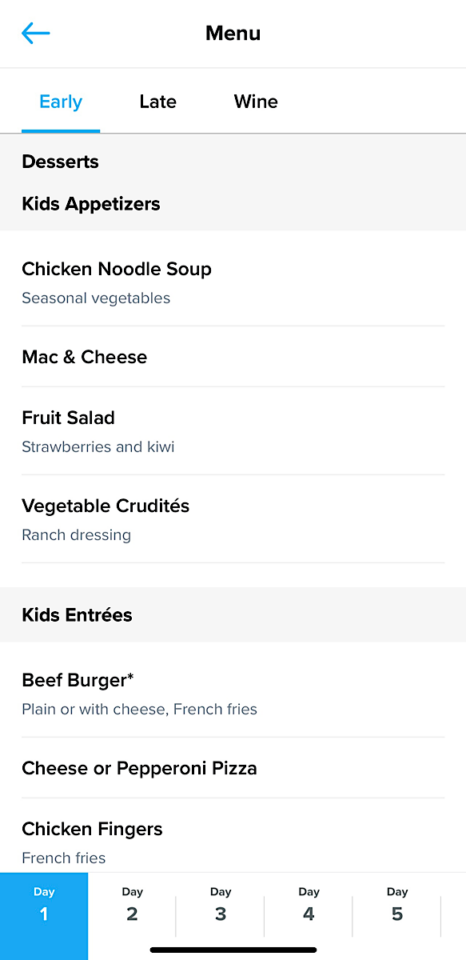This image displays a detailed meal menu page, segmented by various categories visible at the top, such as "Categories," "Early," "Late," and "Wine." Below these main categories, a subsection lists enticing options: "Desserts," "Kids Appetizers," "Chicken Noodle Soup," "Seasonal Vegetables," "Mac and Cheese," "Fruit Salad," "Strawberries and Kiwi," and "Vegetable Crudités with Ranch Dressing." The menu further expands into a "Kids Entrée" section, offering items like "Beef Burger (Plain or with Cheese)," "French Fries," "Cheese or Pepperoni Pizza," and "Chicken Fingers with French Fries."

The screenshot specifically highlights the available meal options for "Day 1" as part of a multi-day meal plan, which extends to "Day 2," "Day 3," "Day 4," and "Day 5." At the bottom of the image, the navigation bar is visible, facilitating seamless interaction with the menu page.